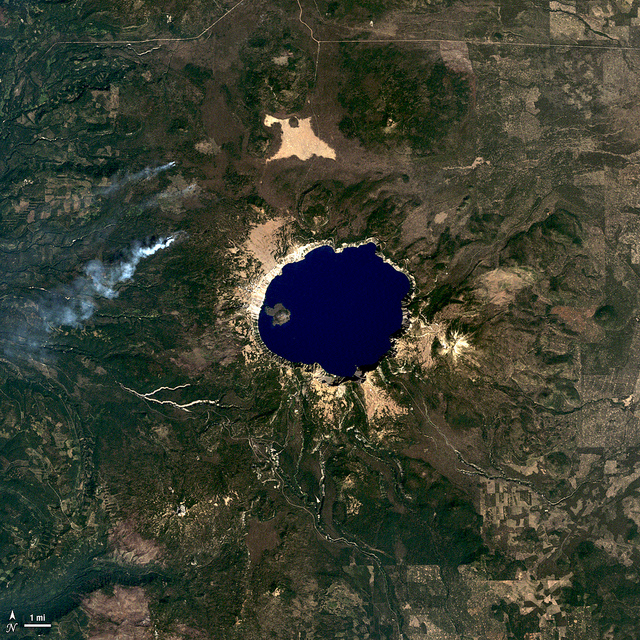This square-shaped photograph, likely taken from a satellite high above the Earth's surface, presents a detailed aerial view of a diverse landscape. Dominating the left side of the image, there is an expanse of lush, green woodland, indicative of large forested areas. Interspersed within this greenery are patches of fire, suggesting active burning in the forest. Rising above the cloud level, the photograph reveals a vibrant blue, roughly circular lake positioned centrally, possibly situated at the summit of a mountain. Surrounding this lake is a lighter, sand-colored beach area, giving way to mountainous terrain on the right side of the image. This mountainous region is more arid, displaying lighter beiges and grays with scant vegetation. Additionally, the bottom left corner of the image contains a scale marker, denoting "north" and measuring up to one mile.